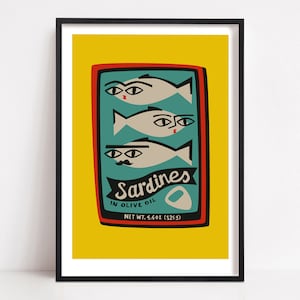In this whimsical and detailed artwork, set against a light gray background, a print is positioned within a black frame. The print itself features a series of vibrant layers: an outer white background, a middle section in bright yellow, followed by a red rectangle, black outline, and finally, an inner light blue area. This composition centers around a humorously depicted sardine can, which stands out with its cartoonish charm. The can is colored predominantly blue and inside it, three sardines swim with amusing details: one sporting a mustache and two bearing feminine features with eyelids and little red mouths. The fish are outlined in black, further enhancing their playful appearance. Accompanying the graphics is text stating "Sardines in Olive Oil" and a somewhat obscured "Net Weight," suggesting it’s 5.6 ounces. This delightful, hand-painted image captures a humorous and creative representation of a sardine can, blending bold colors and charming character designs to bring a smile to any viewer's face.